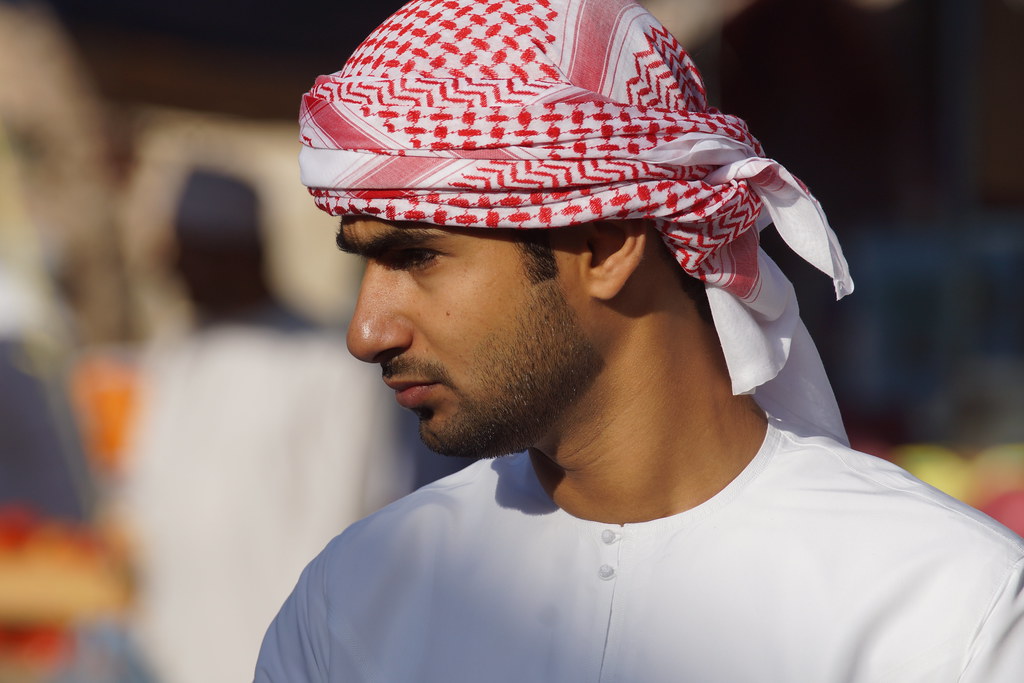The photo captures a young Middle Eastern Muslim man in his late teens to early twenties, dressed in traditional attire. He wears a red and white patterned scarf, distinct with zigzag lines and small red squares, wrapped around his head. His toned skin and neatly trimmed, closely cropped beard frame his medium-complexioned face which is partially shadowed by his head wrap. The man dons a plain white robe with a rounded collar, buttoned up to the top. Facing the camera but looking to his right, he maintains a composed expression. The scene is set on a sunny day, likely at an outdoor market or a busy street, though the background remains blurred and indistinct, hinting at the presence of another figure and possibly vibrant market stalls. The sun casts a hard shadow over his face and neck, highlighting the brightness of day.